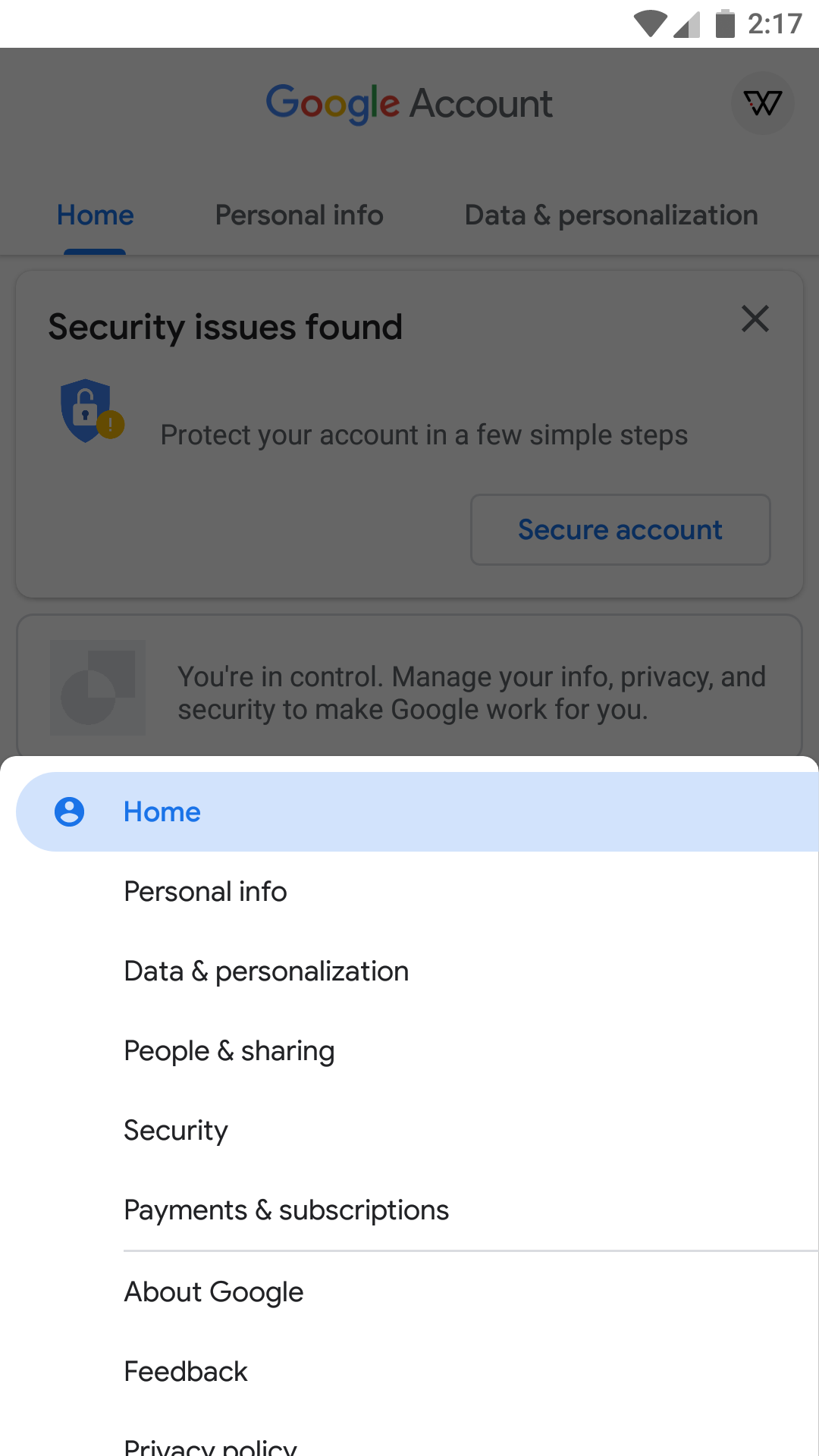The image displays the Google Account section on a mobile device. The upper half of the screen features a white background with the Google logo to the left and the word "Account" next to it. In the top-right corner, there's a profile picture representing the user's account.

Beneath this header are tabs labeled "Home," "Personal Info," "Data & Personalization," indicating navigation options within the account settings. A prominent white box on the screen alerts the user to security issues, featuring a shield with a white lock symbol and a yellow exclamation mark. The message reads "Protect your account in a few simple steps," accompanied by a button to secure the account.

Below this section, a pop-up screen overlays the page with various navigation tabs including "Home," "Personal Info," "Data & Personalization," "People & Sharing," "Security," "Payments & Subscriptions," "About," "Feedback," and "Privacy Policy." The "Home" tab is highlighted in light blue, indicating it is currently selected. The overall layout is clean and user-friendly, guiding the user through important security and account management features.